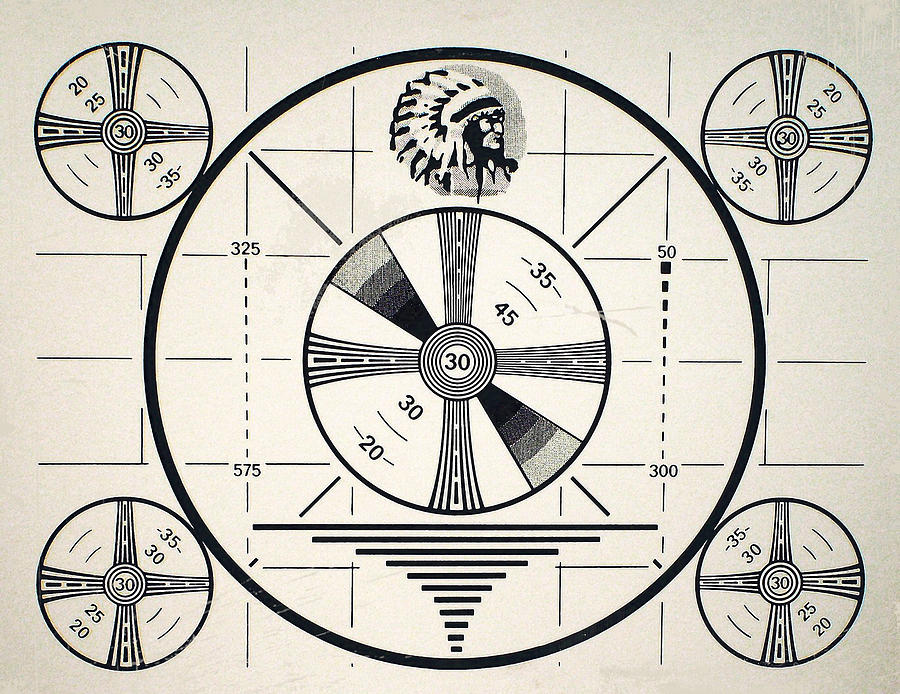The image appears to be a black-and-white television test pattern from the 1950s. It features a central black circle outlined with a grid-like square pattern. Within the central circle is a detailed drawing of a Native American chief in a headdress, gazing into the distance. Concentric circles within this central circle contain various lines and numbers including 35, 45, 30, 30, and 20. Four identical circular discs are positioned in each corner of the image, each displaying a series of numbers: 20, 25, 30, and 35, reminiscent of vinyl records. All numbers are arranged with lines extending outward to the black rim of the main circle, adding to the geometric complexity of the design. The entire image is monochromatic, utilizing only shades of black, white, and gray, set against a cream-colored background.